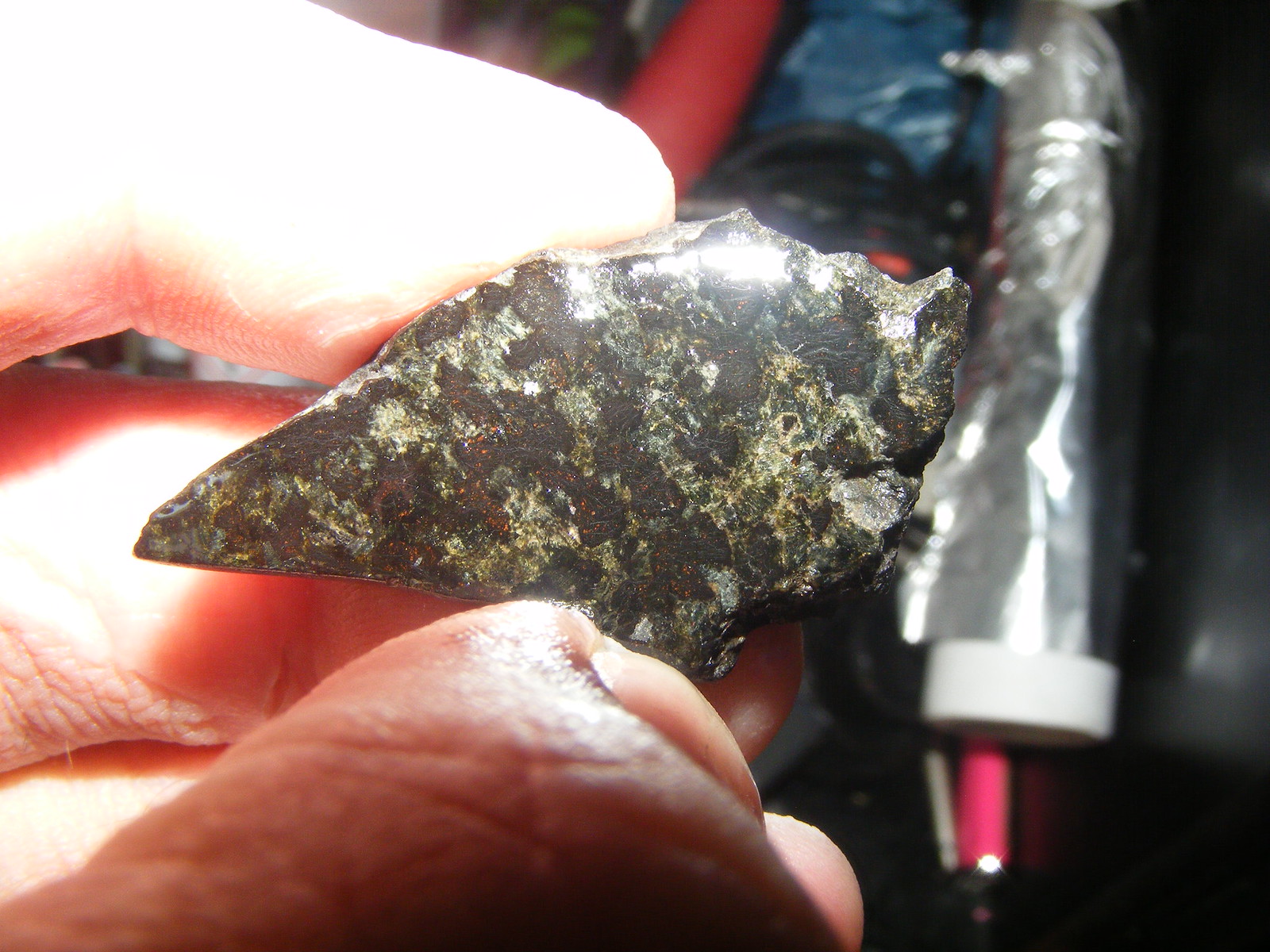The image is an extreme close-up photograph of a man's fingers holding a jagged piece of stone, reminiscent of an arrowhead in shape. The stone, predominantly black and green with hints of gold, white, gray, and possibly red, is held at its blunted right end with its pointy left end protruding out. The surface of the stone is shiny and smooth, reflecting bright light that hits it. The man's fingers, appearing sturdy and indicative of a Caucasian male, are lit by the same bright light, making their texture and details prominent. In the slightly blurred background to the right, there are rolls of paper in various shiny colors – silver, blue, and pink, adding a touch of contrast to the focused stone and fingers.